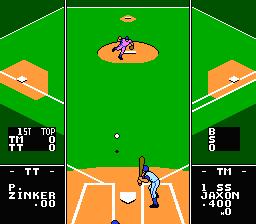A nostalgic screenshot captures the essence of an 8-bit baseball video game. The simple yet charming graphics reveal all four bases on a vividly green field. At home plate stands a determined batter poised to swing at an approaching ball, with its shadow clearly visible below. The pitcher is captured mid-throw, his arm extended in a classic pitching motion. 

The screen is framed with essential game information; black squares to the sides display scores, while player statistics enhance the narrative. A name is showcased on the left, and on the right, another name accompanied by the player’s batting average. 

Above these, a classic baseball graphic indicates the game's progress—situtated in the top of the first inning. The score is tied at 0 for both teams, labeled "TM" and "TT". The simplicity and distinctive 8-bit design of this image evoke a sense of retro gaming nostalgia.